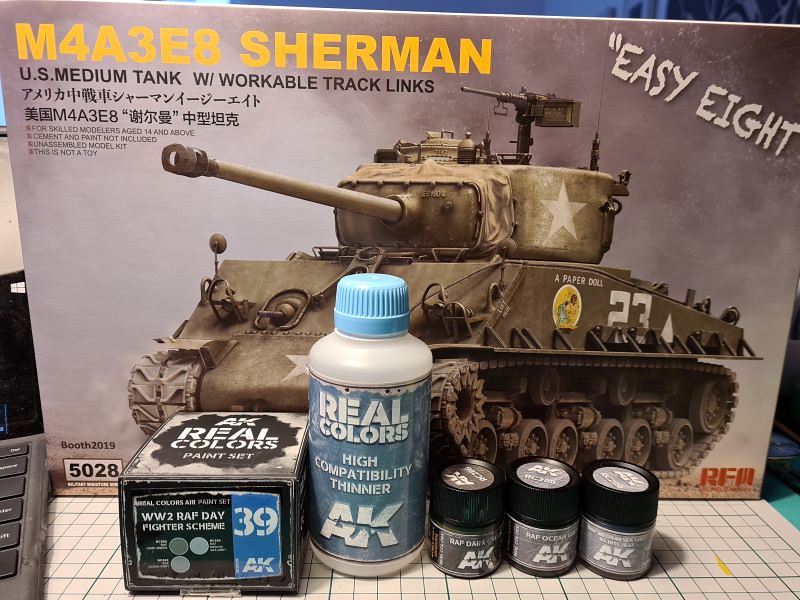The image depicts the front of a model kit box for an M4A3E8 Sherman tank. The box is standing upright on a surface with a craft metal grid. At the top left of the box, in large bold gold text, it reads "M4A3E8 Sherman." Below in black text, it states "U.S. medium tank with workable track links," followed by sentences in Chinese and Japanese characters, translating to "American M4A3E8." Additionally, it specifies "For skilled modelers aged 14 and above" and notes that "cement and paint are included." 

A diagonal inscription at the top right reads "EZ-8." The central image features a painted side-angle view of the tank, showcasing its turret, machine gun on top, front cannon, side tracks, and engine at the rear. The tank is rendered in green with white stars on both the side and front. The number "23" and the phrase "A Paper Doll" appear in white on the tank's side. 

Adjacent to the box on the left is a smaller rectangular box labeled "AK Real Colors paint set, WW2 RAF Day Fighter scheme," in white text on a black background. Accompanying the paint set are a clear plastic bottle labeled "Real Colors High Compatibility Thinner," and three small cylindrical paint pots labeled "RAF Dark," "RAF Ocean," and an uncertain third color, each with black caps and white text.

In the background, details like graph paper, a calculator with gray buttons, and a gray device with a black screen displaying a Windows logo are visible. Overall, the detailed presentation emphasizes the comprehensive nature of the model kit and the associated painting supplies, set against a mix of subdued green and gray tones.